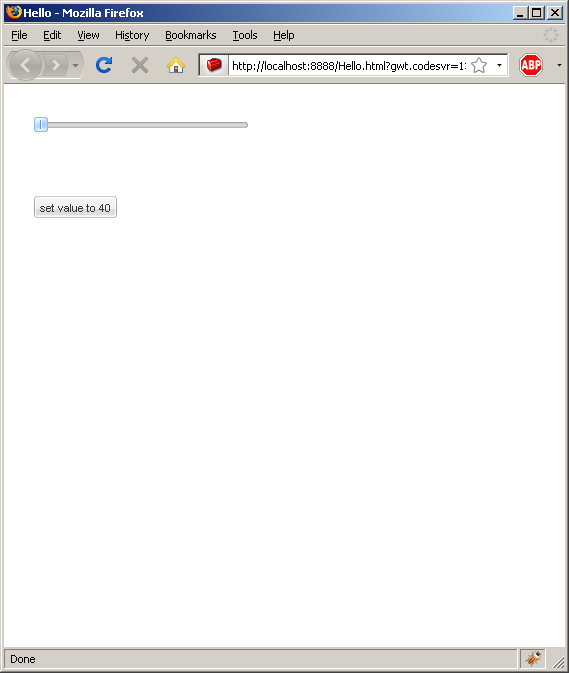This image is a screenshot of a computer display showing a web browser, specifically Mozilla Firefox, featuring a predominantly white background with minimal content. At the very top of the screenshot, there is a blue bar with the text "Hello, Mozilla Firefox." Below this blue bar, the usual browser menu options are visible, including "File," "Edit," "View," "History," "Bookmarks," "Tools," and "Help."

Further down, there is a navigation toolbar with left and right arrow buttons; the left arrow is emphasized with a bold circle around it, indicating it may have been recently used. Additionally, several icons are present: a blue circular arrow symbol (likely the refresh button), a gray X (possibly for stopping the loading process), and a house icon for the homepage. The address bar shows the URL "http://localhost:8888/hello" and some other indistinct text.

In the main white area of the screen, at the upper left, there is a gray bar that resembles a volume control, with a blue square on its left side. Directly beneath this bar, a small gray rectangle contains the black text "Set value: 240."

Finally, at the very bottom of the screen, there is a gray status bar, with the word "Done" displayed in black text in the bottom left corner.